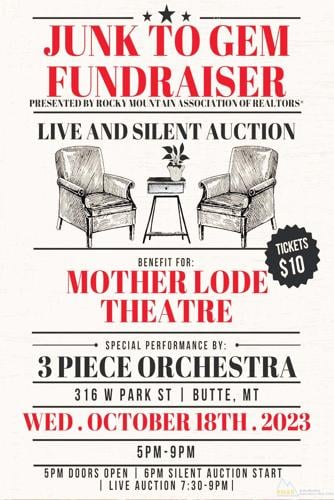The vertical poster features a solid white background, with some off-white coloring at the very top. It prominently displays "JUNK TO GEM FUNDRAISER" in all caps red letters at the top center, flanked by three small black stars above it. Below this title, "PRESENTED BY ROCKY MOUNTAIN ASSOCIATION OF REALTORS" is written in smaller, all caps black letters. A horizontal black line separates this section from the next.

The next part announces "LIVE AND SILENT AUCTION" in black text, followed by an image depicting two armchairs and a small table with a potted plant between them. Beneath this image, "BENEFIT FOR MOTHER LODE THEATER" is displayed, where "MOTHER LODE THEATER" is in all caps red letters with "BENEFIT FOR" in black. To the right of this text, a black circular bubble with white letters states "TICKETS $10."

Another horizontal black line divides the content above from the upcoming details. The text underneath reads "SPECIAL PERFORMANCE BY THREE PIECE ORCHESTRA," with "THREE PIECE ORCHESTRA" in all caps black letters. The address "316 West Park Street, Butte, Montana" is provided in black text, followed by the event date and time in red letters: "WEDNESDAY, OCTOBER 18th, 2023," with the event running from "5 P.M. to 9 P.M." Further breakdown states that doors open at 5 P.M., the silent auction starts at 6 P.M., and the live auction runs from 7:30 P.M. to 9 P.M.